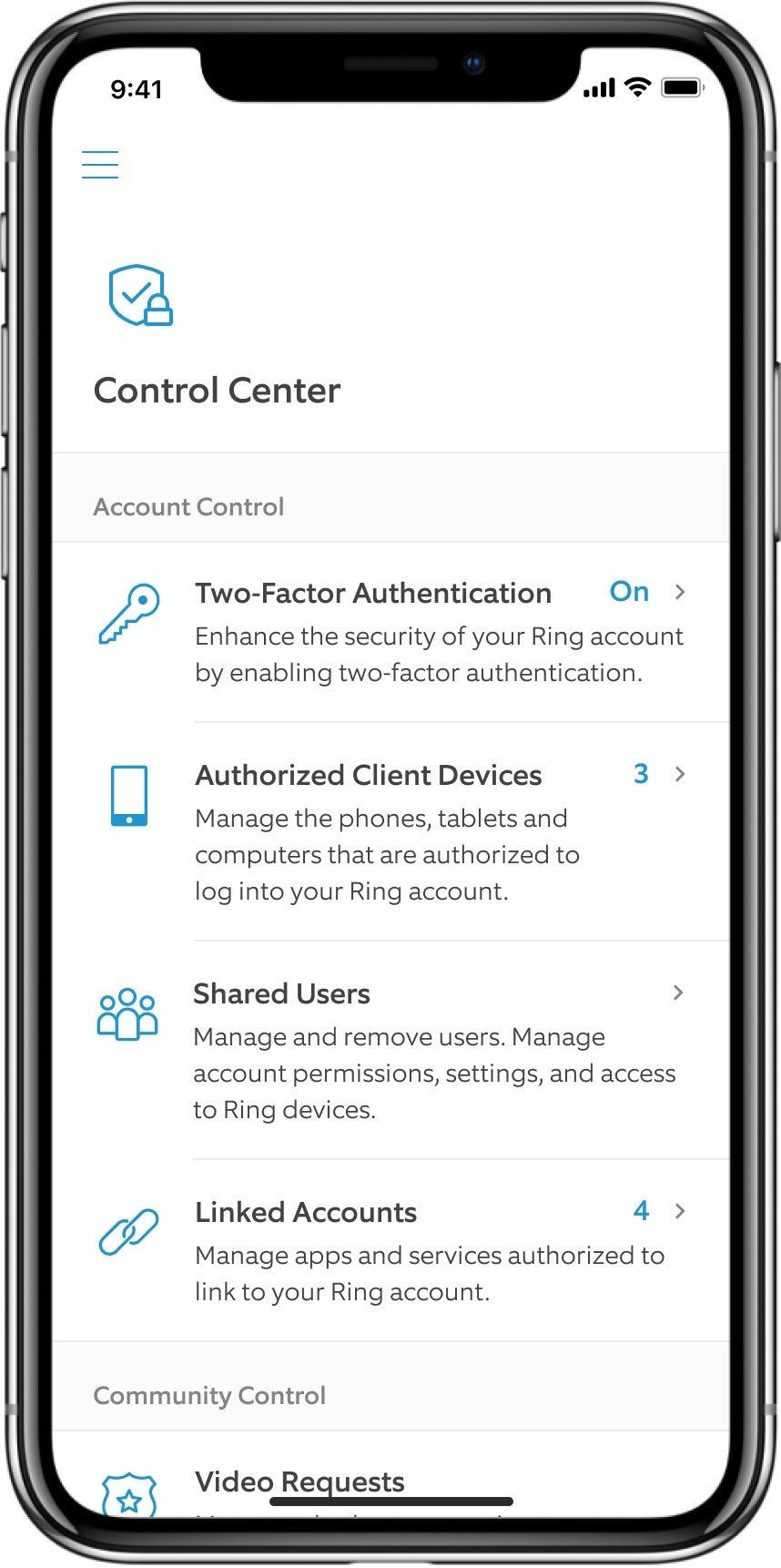Screenshot of a mobile phone’s control center interface for Ring account security settings. The interface prominently features a shield icon with a checkmark indicating active security. The "Account Control" section displays various security options:

- **Two-Factor Authentication**: Active protection with the ability to authorize client devices. A blue number three indicates the devices currently authorized.
- **Manage Devices**: Allows management of phones, tablets, and computers that are authorized for Ring account access.
- **Shared Users**: Includes an icon of multiple people, indicating the option to manage and remove users.
- **Account Permissions**: Provides settings to manage account permissions and access to Ring devices.
- **Linked Accounts**: An area to view and manage linked accounts.
- **Community Control**: Includes options like video requests, providing additional security and community management features.